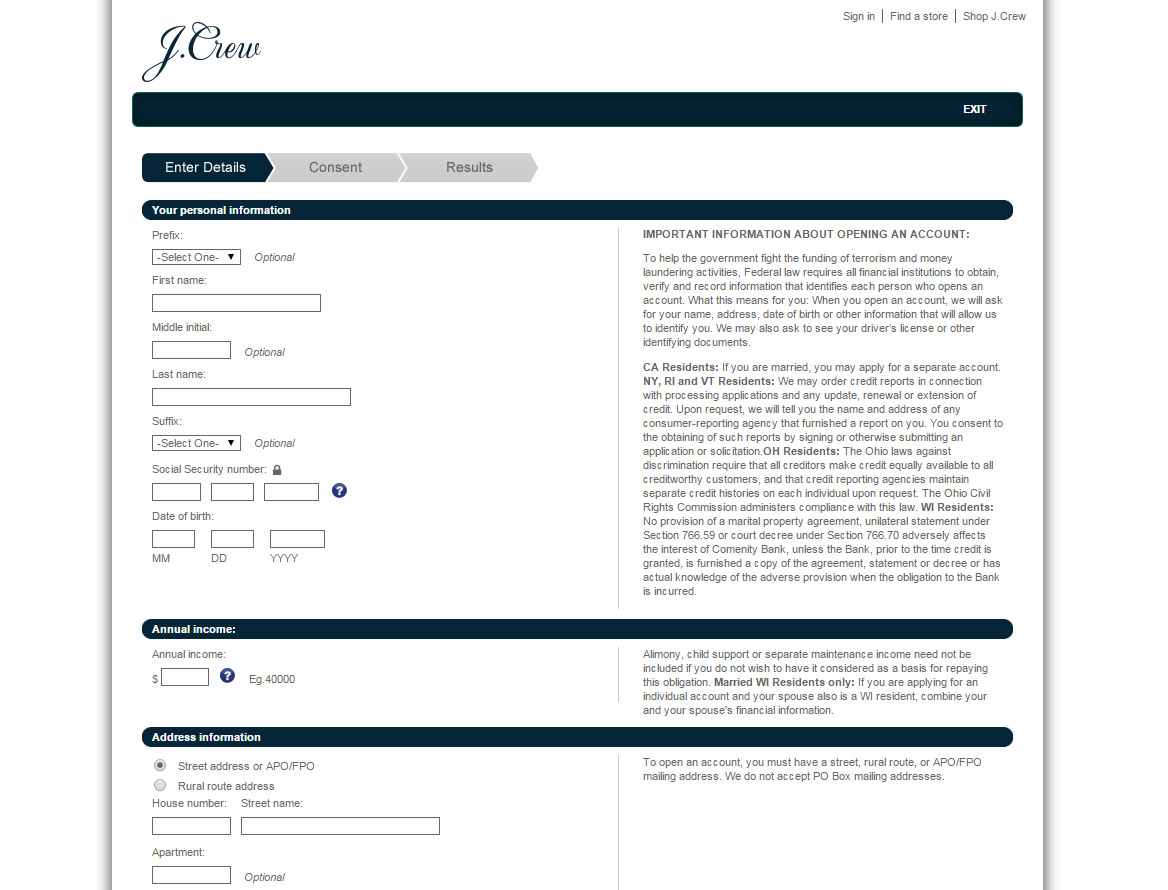This image is a screenshot from the J.Crew website, showing an application form for opening an account or applying for a credit card. The page has a clean, white background with black text. In the upper left corner, the J.Crew logo is prominently displayed. On the right side of the header, there are links for "Sign In," "Find a Store," and "Shop J.Crew.”

Below the header, a black border frames the application form, which is currently on the "Inner Details" screen, part of a multi-step process also including "Consent" and "Results." The section is titled "Your Personal Information."

Within this section, there is a dropdown for selecting a prefix (optional), followed by input fields for the first name, middle initial (optional), and last name. There is also a dropdown menu for a suffix (optional). The form requests a Social Security number and date of birth. Further down, it asks for the applicant's annual income and address information. A checkbox for the street address appears to have been selected.

On the right side of the screen, there is a sidebar containing important information about opening an account. The comprehensive layout and the specific data being requested suggest that the user is likely in the process of applying for a J.Crew account or credit card.